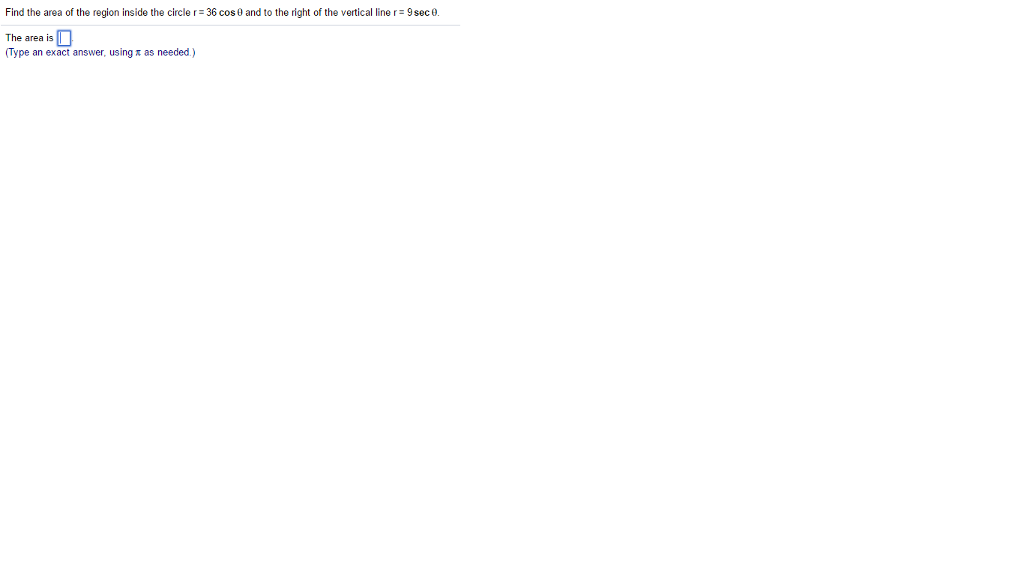This is a screenshot of a math question from an online resource, featuring a predominantly white background with considerable negative space on the bottom and right. The main content is concentrated in the top-left section of the image. The first line, placed in the very top-left corner, contains the question written in small, dark gray or black sans-serif text. The question reads: "Find the area of the region inside the circle \( R = 36 \cos \theta \) and to the right of the vertical line \( R = 9 \sec \theta \)." Below this question is a thin, light gray line that runs the entire width of the question, acting as a separator between the question and the answer area. 

In the answer area, there are two textual lines. The first line, in the same sans-serif font as the question, states "The area is," followed by a text box outlined with a medium blue glow, containing a blinking vertical cursor. Below this, in slightly blue text and enclosed in parentheses, the instruction reads: "Type an exact answer using x as needed."